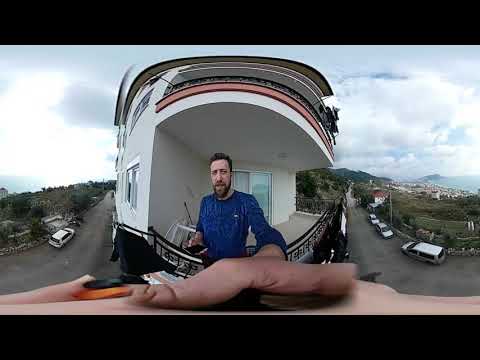In the fisheye-lens-distorted image capturing a wide-angle view, a bearded white man with brown hair, wearing a blue long-sleeve shirt, stands on the second-floor balcony of a white building, likely a motel or apartment. His right hand hovers just above his stomach while his left hand reaches forward, magnified and distorted by the camera lens. Behind him is a black railing, draped with a black cloth on the left side, and a blue-tinted sliding glass door. Above, the building's trim is intricately colored with white, orange, and brown, topped with a silver section. 

The surrounding environment showcases two crisscrossing gray streets. To the left, a lone white car drives past green vegetation and trees. The right street hosts three silver cars parked along the curb, with a white house with an orange roof in the distance. The background features a town skyline far off, under a sky painted with hues of white and gray clouds, evoking a serene and somewhat tropical ambiance.